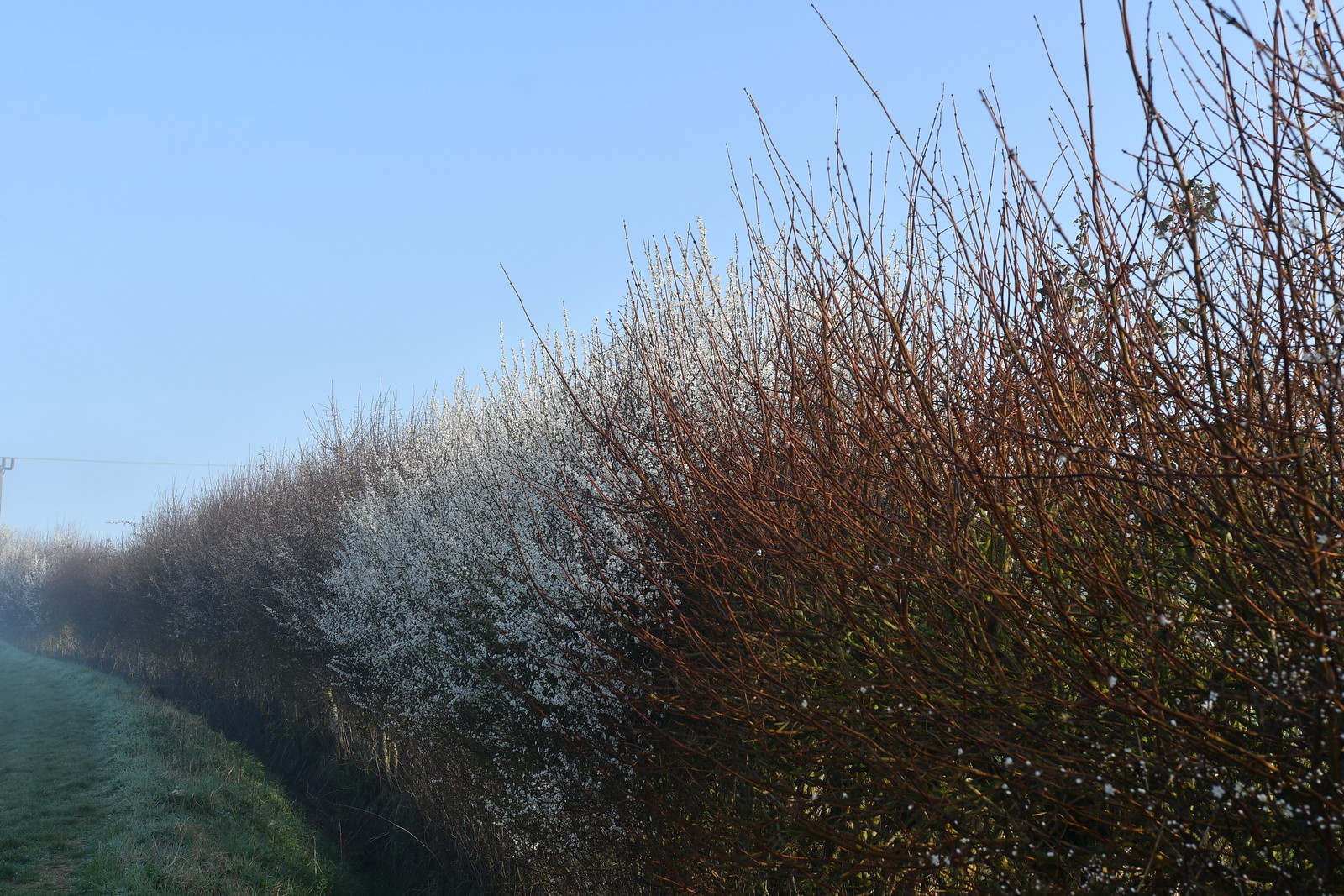The photograph captures a winter or late autumn scene dominated by a line of wild, sparsely foliated bushes curving slightly to the left. Along the right side, the bushes present mostly bare branches with some dead brown leaves. In contrast, the bushes in the middle of the image display branches tipped with white, cotton-like blooms, giving the appearance of either frost or seeding. Above the bushes, the sky is a clear, light blue, indicating early morning light. The lower left corner shows a patch of green grass, hinting at a narrow stream of water possibly running through the area. The distant background features faint outlines of power lines, suggesting the presence of human activity in an otherwise natural landscape.